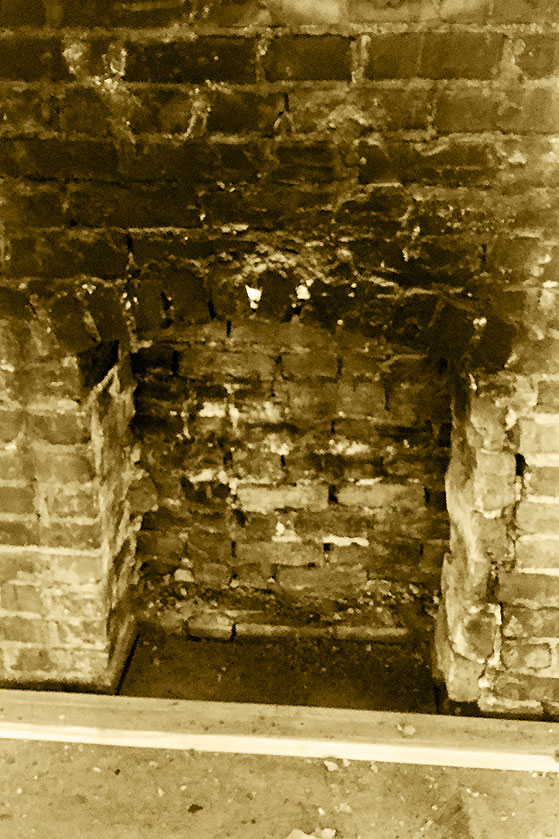The image depicts a disused and weathered fireplace positioned centrally within the frame, set against a backdrop of a brick wall. The overall color palette is heavily tinted with high saturation, creating a yellowish or rare shade of brown hue, though it predominantly varies between black, white, and shades of gray, with hints of tan. The fireplace appears neglected, featuring a wooden or marble beam at its base and a concrete floor littered with dirt and rocks. The bricks forming the upper section of the fireplace are darker, possibly suggesting burn marks or extensive soot accumulation, while the inside of the fireplace, though somewhat charred, is not as severely burnt. There is a noticeable contrast in brick shades, adding to the sense of deterioration and disuse. The setting seems to be indoors, likely within an old or poorly maintained house.